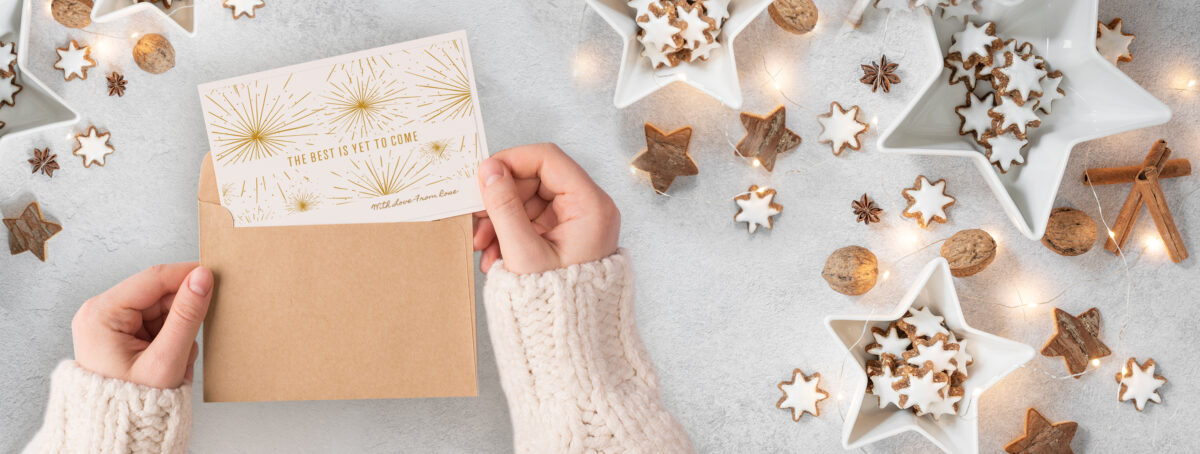In this overhead shot, a pair of hands in a white knit sweater are seen delicately pulling a white invitation card from a light brown envelope. The invitation, adorned with elegant gold font, reads "The best is yet to come". Spread across the white tabletop are various decorations creating a festive scene. Star-shaped white bowls hold star-shaped cookies with white icing, scattered around the table are more star cookies, walnuts, and cinnamon sticks. Fairy lights are artfully draped among the items, giving a holiday-esque ambiance. The tabletop is sprinkled with assorted brown buttons and stars of different sizes and colors, adding a whimsical touch to the composition. The light brown envelope and associated festive decor suggest a warm, inviting atmosphere.